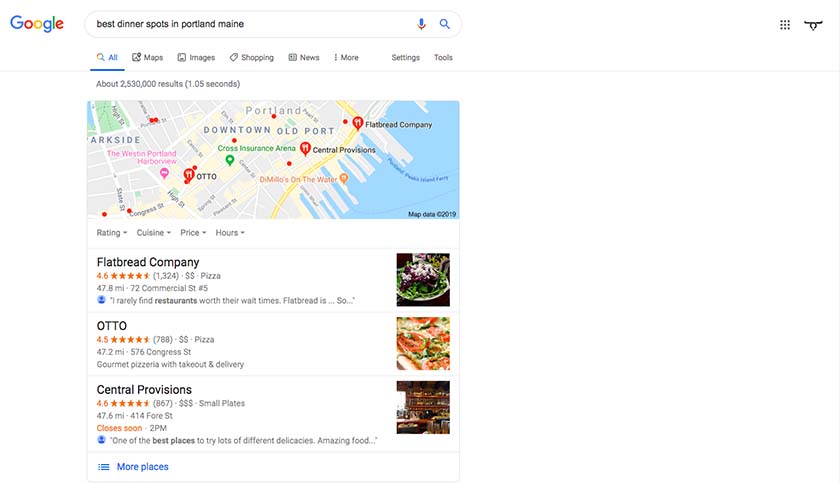Here is the cleaned-up and detailed caption for the described image:

---

The image captures a Google search results page with a clean white background. In the top left corner, the standard vibrant Google logo is displayed prominently. To its right, the search bar contains the query "best dinner spots in Portland, Maine." Inside the search bar, to the right, are a microphone icon and a magnifying glass icon. Further to the right of the search bar, there are three vertical dots followed by a grid of 3x3 dots and a badge.

Below the search bar, a series of tabs are aligned horizontally. Each tab sports its own distinct icon: "All" with a magnifying glass, "Maps" with a map icon, "Images" with a standard image icon, "Shopping" with a price tag icon, "News" with a newspaper icon, and "More" accompanied by three dots. Adjacent to these tabs are the options for "Settings" and "Tools."

The search yielded approximately 2,530,000 results, displayed in 1.05 seconds. Below this summary, there is a map highlighting the search area.

Under the map, several filter options appear in gray text, such as "Rating," "Cuisine," "Price," and "Hours."

The first result showcases "Flatbread Company." It is shown in black text, boasting a rating of 4.5 stars from 1,324 reviews. Represented by dollar signs indicating its price range ($$), it serves pizza and is located 47.8 miles away at 72 Commercial St, #5. A brief review from a default profile icon reads, "I rarely find restaurants worth the wait times. Flatbread is..." with an image of food accompanying it.

The second result features "OTTO" in uppercase letters, also rated 4.5 stars from 768 reviews. With double dollar signs ($$), this pizzeria offers both takeout and delivery options and is located 47.2 miles away at 576 Congress Street. A description below reads, "Gourmet pizzeria with takeout and delivery," alongside a close-up photo of pizza.

The third result is "Central Provisions," with a 4.5-star rating from 967 reviews. This restaurant has a price range denoted by three dollar signs ($$$) and offers small plates. Located 47.6 miles away at 414 4th St, it is marked with orange text indicating it is "Closing Soon, 2 PM." A review states, "One of the best places to try lots of different delicacies. Amazing food," paired with an image resembling a library-like, brown interior.

Beneath these entries, there is a section titled "More places," inviting users to click a link for additional options.

---